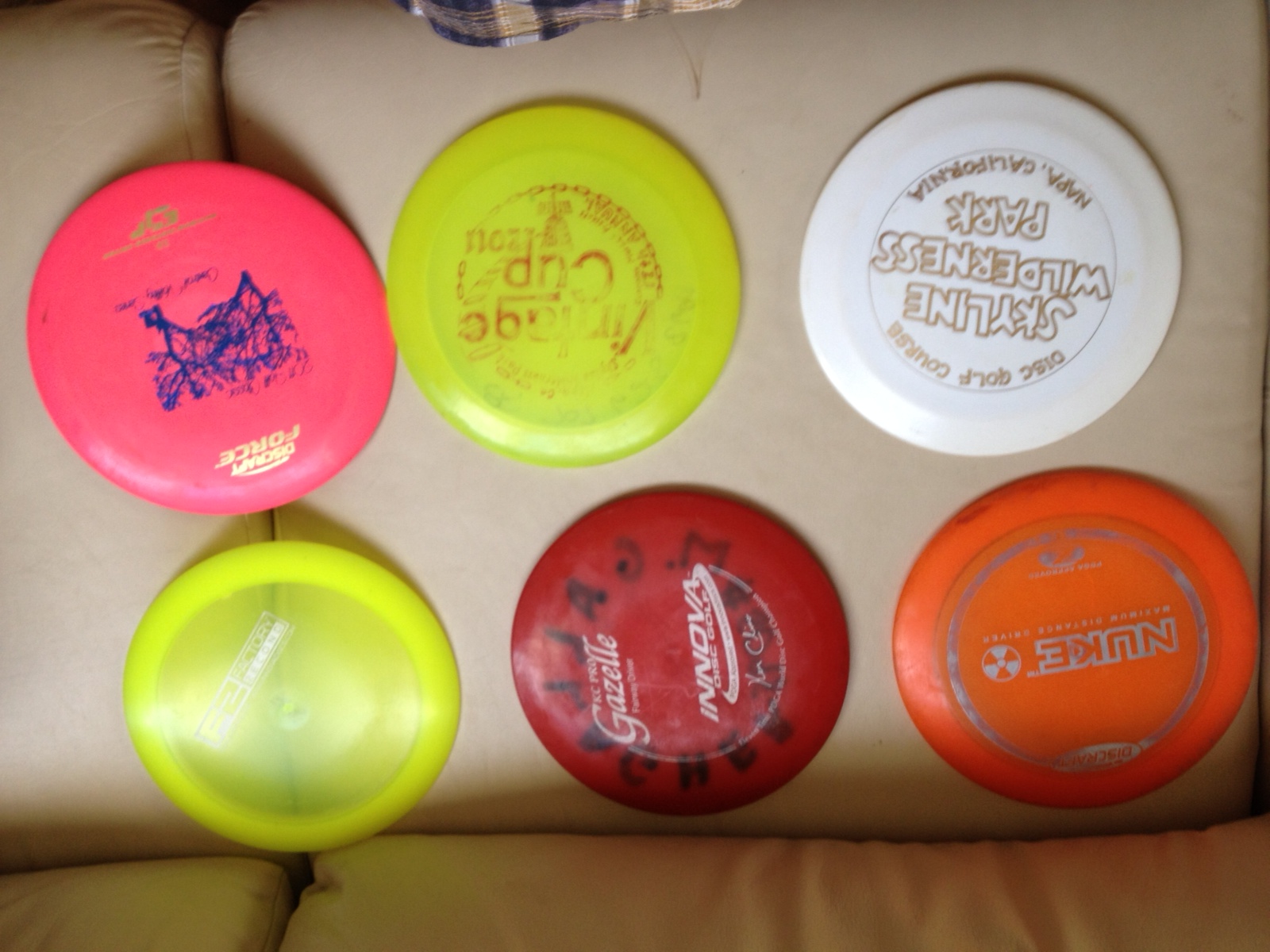The photograph showcases a top-down perspective of six frisbees arranged in a neatly spaced display pattern on a beige faux leather couch. The frisbees are divided into two rows, with three on the bottom and three on the top. From bottom right to left, the colors of the frisbees are: yellow with faded writing, red and white with a black magic marker inscription, and orange and white with the word “Nuke” and a small Nuke icon. From top right to left, the colors are: pink and gold, yellow and red, and white with black lettering that reads “Skyline Wilderness Park.” Additional decipherable text includes “Innova” and “Gazelle,” though much of the writing is faded or unclear. The image is composed from an angle standing over the couch, capturing the frisbees laid out on two separate long cushions.